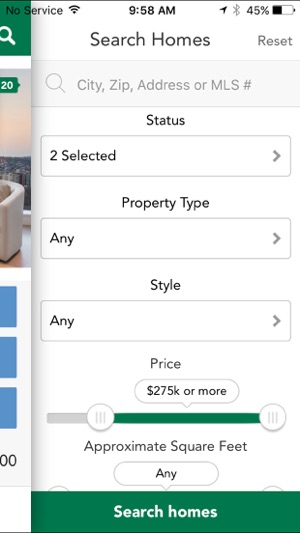The image displays a smartphone screen where someone is searching for a home to buy. In the top left corner, "No Service" is shown in black font. Adjacent to it is the Wi-Fi symbol, indicating a full network. Centered at the top is the time, 9:58 a.m. On the top right, icons for location services (an arrow), Bluetooth, and a battery status at 45% are visible.

Below, the screen's background is predominantly white. At the top of this section, "Search Homes" is written in light black or dark gray font, and to its right is the word "Reset" in gray font. Beneath, there is a gray search bar with a magnifying glass icon, suggesting inputs like city, zip, address, or MLS number.  

Further down, the interface lists options such as "Status" with a selected option, "Property Type" with an accompanying right arrow for selection, and "Style" with another right arrow. At the bottom, there is a price slider set to $275,000 or more, and an "Approximate Square Feet" option currently set to "Any." Finally, a green button labeled "Search Homes" is prominently displayed for executing the search.